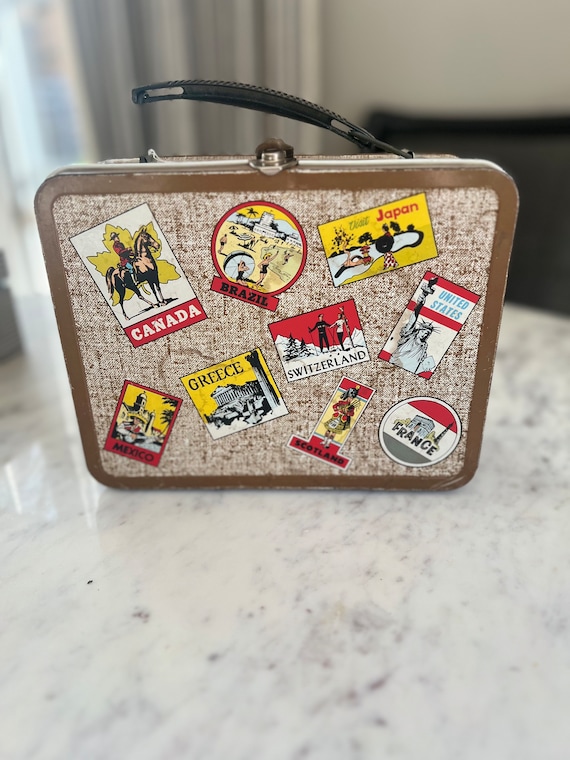This photograph, taken in portrait orientation, showcases a vintage metal lunchbox resembling a thin, small suitcase with rounded corners. The box, positioned upright with the lid facing the viewer, is adorned with travel stickers from various countries including Canada, Brazil, Japan, the United States, Switzerland, Greece, Mexico, Scotland, and France. These stickers, showcasing famous landmarks, are arranged in a random pattern and feature simple colors of red, blue, black, and white.

The lunchbox has a distinctive dark brown trim around the perimeter of the lid and a tweed-like texture in white and brown on its surface. A broken plastic handle, black in color, is located at the top, and a partially raised silver clasp lock is visible in the middle. The detailed background reveals an out-of-focus living room, while the lunchbox rests on a light-colored marble table with gray speckles. The overall style of the photo falls under photographic representationalism, realism, and product photography.